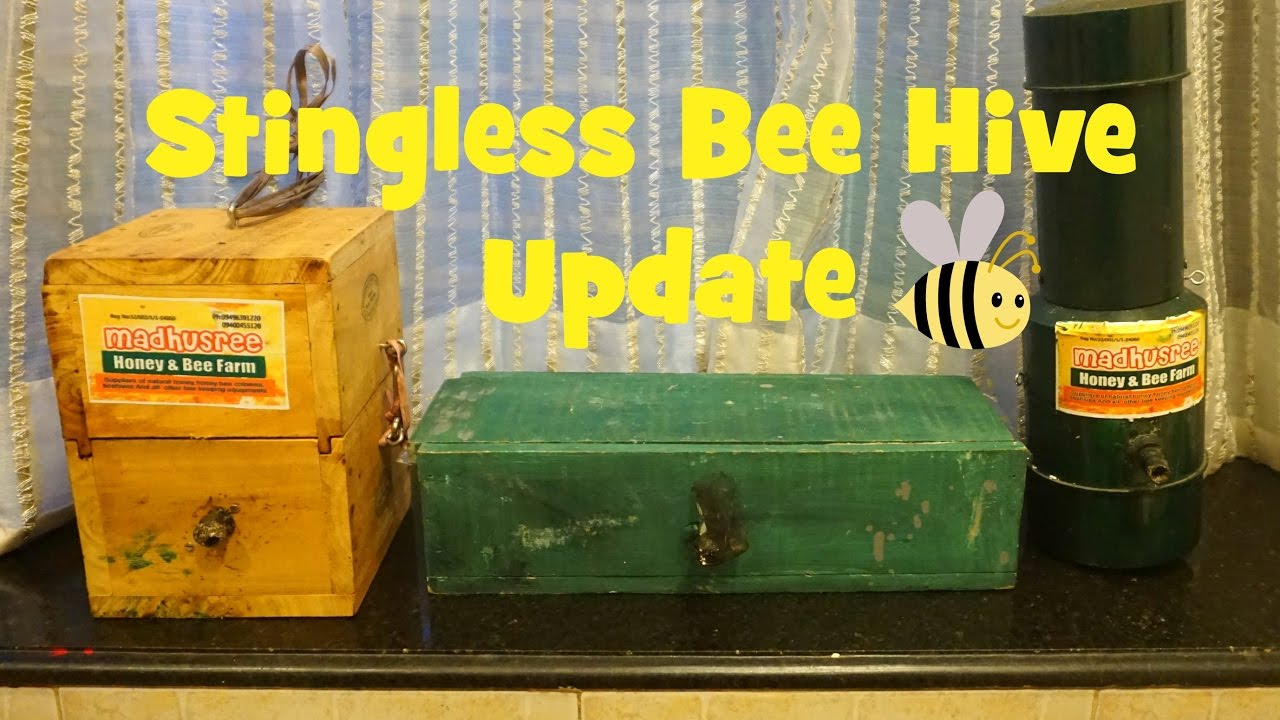The image appears to be an indoor color photograph, likely used as cover art for a YouTube video or a banner from a website promoting a honey bee farm. On a countertop, there are various bee-related items neatly arranged. To the left, there is a wooden bee box with a sticker labeled "Mad Huzzary Honey and Bee Farm." This box features a latch and looks functional. In the center, an old, green-painted wooden box, also with a latch, is set in a rectangular shape and appears quite aged. On the far right, there's a black canister, possibly a bee smoker, also labeled with the "Mad Huzzary Honey and Bee Farm" sticker. 

The backdrop consists of a fancy, sheer curtain resembling a shower curtain, with horizontal stitches adding a subtle touch of elegance to the scene. Additionally, the entire image features a cartoony yellow text overlay reading "Stingless Beehive Update," with a small cartoon bee at the end of the phrase, emphasizing the theme. The collection of items and the overall setup suggests a promotional image designed to inform and engage viewers about the bee farm activities.